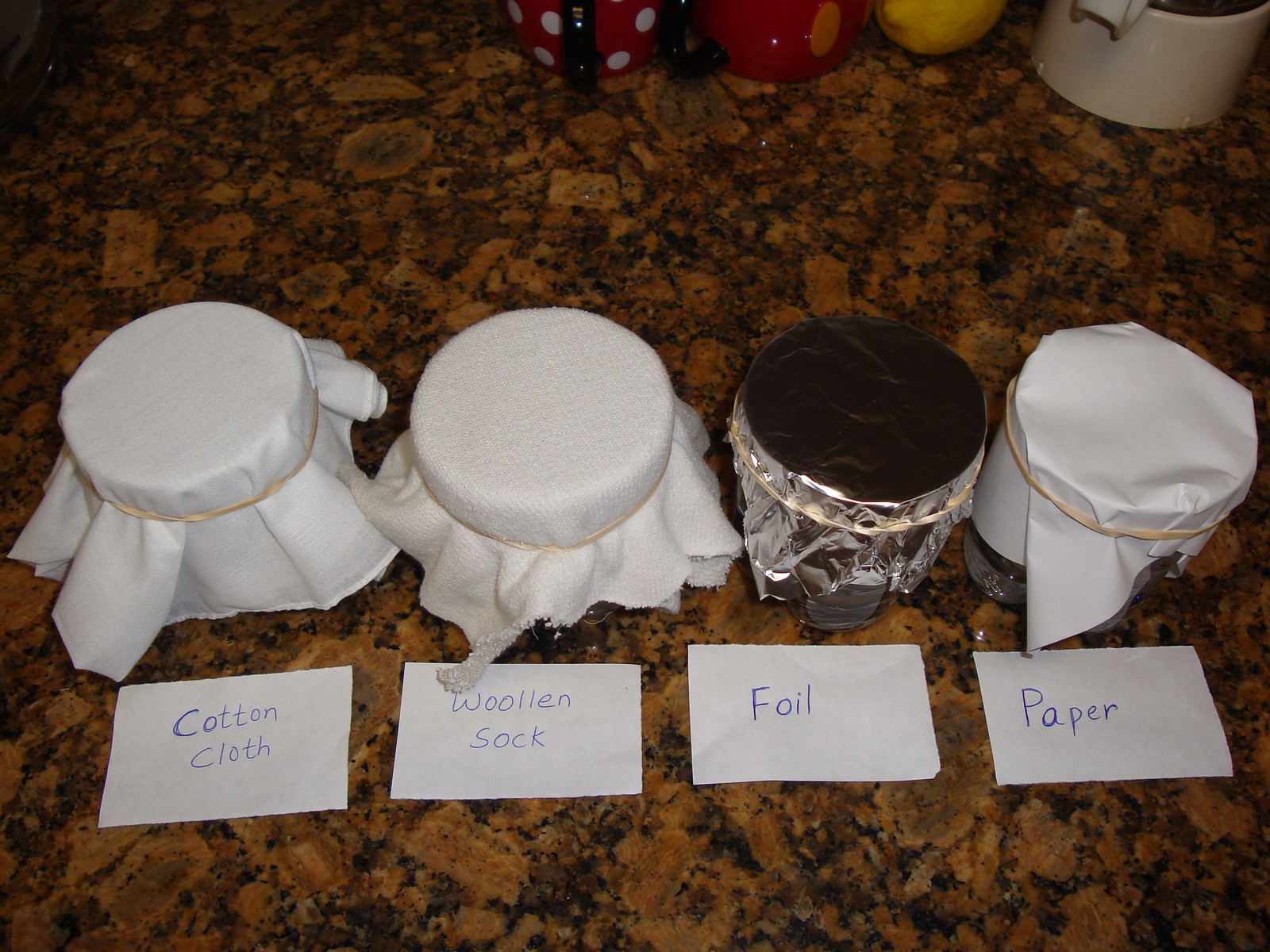The photograph captures a close-up view of four small glass jars, each approximately the size of a short drinking glass or small coffee cup, arranged in a row on a dark brown, coppery granite kitchen countertop. Each jar is covered with a different material, all secured in place with rubber bands. From left to right, the first jar is covered with a white cotton cloth, labeled "cotton cloth" in blue pen on a small piece of paper in front of it. The second jar is topped with a white woolen sock, labeled "woolen sock." The third jar is sealed with aluminum foil, labeled "foil," distinguished by its silver color. The last jar is covered with a white sheet of paper, labeled "paper." In the background, various colored mugs are partially visible, adding to the kitchen setting.